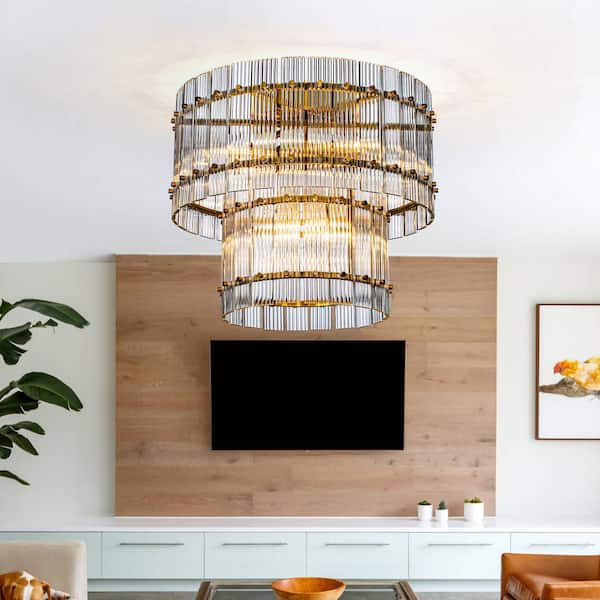The image showcases a stylish and upscale living room. Central to the scene is a flat-screen TV mounted on a light wood-paneled accent wall, with the surrounding walls painted a subtle off-white. Directly above, the white ceiling features a striking, ornate chandelier composed of two cylindrical, gold-colored structures—a larger one above and a smaller one hanging below, both emitting a warm glow. Below the TV, there are sleek, white cabinets and a white bench-like shelf.

On the bottom left corner, a cream-colored couch arm is visible, while the bottom right corner reveals a brown leather chair. A glass-topped coffee table sits between them, adorned with a brown bowl. At the center left, a dark green leafy house plant adds a touch of nature to the room. The floor appears to have a modern gray tone, complementing the room's sophisticated atmosphere. There's also a white-trimmed picture on the right wall, featuring gold and brown elements, contributing to the overall elegant décor.